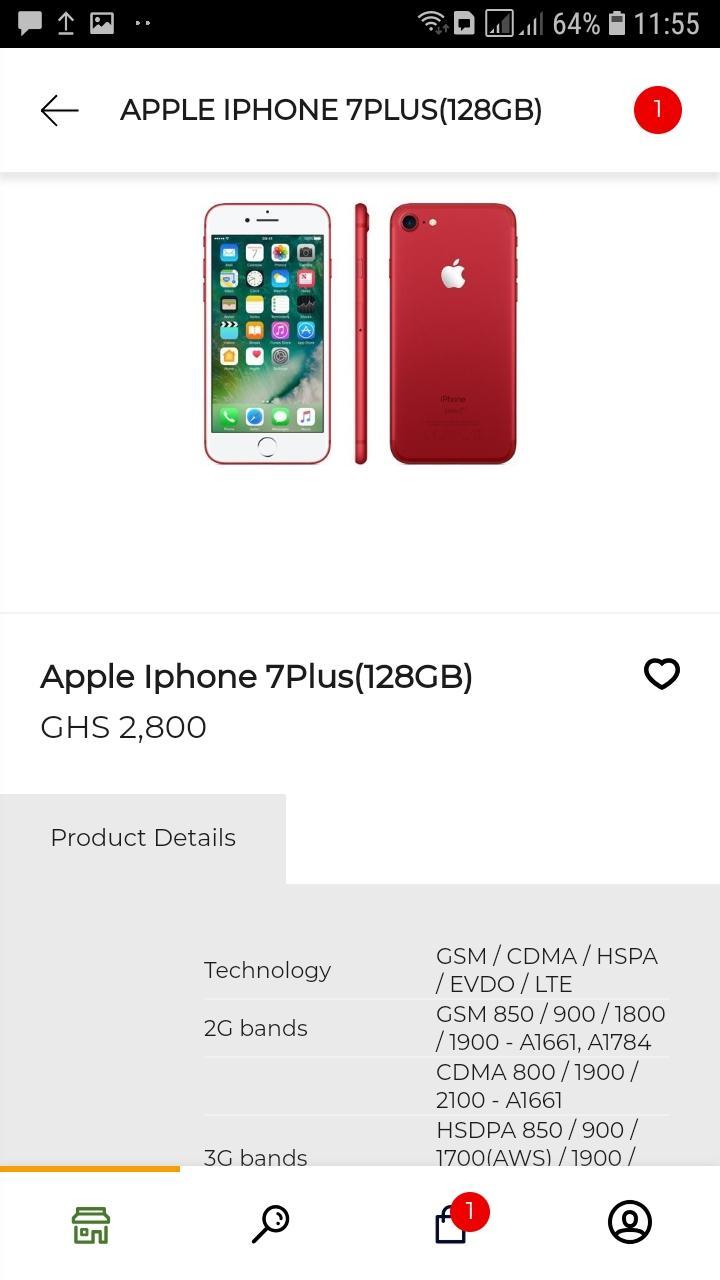The image displays a detailed product listing of an Apple iPhone 7 Plus with 120GB storage. The screenshot appears to have been taken on a smartphone, as indicated by the black status bar at the top, which shows full Wi-Fi signal, a 64% battery life, and the time as 11:55. 

Prominently featured in the visual are several elements:
- The left side of the screen displays a back arrow.
- The main section showcases a red Apple iPhone 7 Plus. The device is specified to have 120GB of storage.
- The background is light, which enhances the visibility of the red iPhone.
- A red circle highlights certain aspects of the product.
- Some tech specifications include the phone’s compatibility with various technologies: GSM, CDMA, EVDO, LTE. The frequency bands listed are GSM (850, 900, 2200, 2600), CDMA (800, 1900, 2100), and HSDPA (515, 900, 1700 AWS, 1900).

Additional interface features visible:
- A magnifying glass icon, suggesting a search function.
- A shopping bag icon, likely indicating a cart or purchase option.

The entire scene unmistakably looks like a snippet from an online shopping platform, where product details such as price (GHS 2800) and technical specifications are provided.